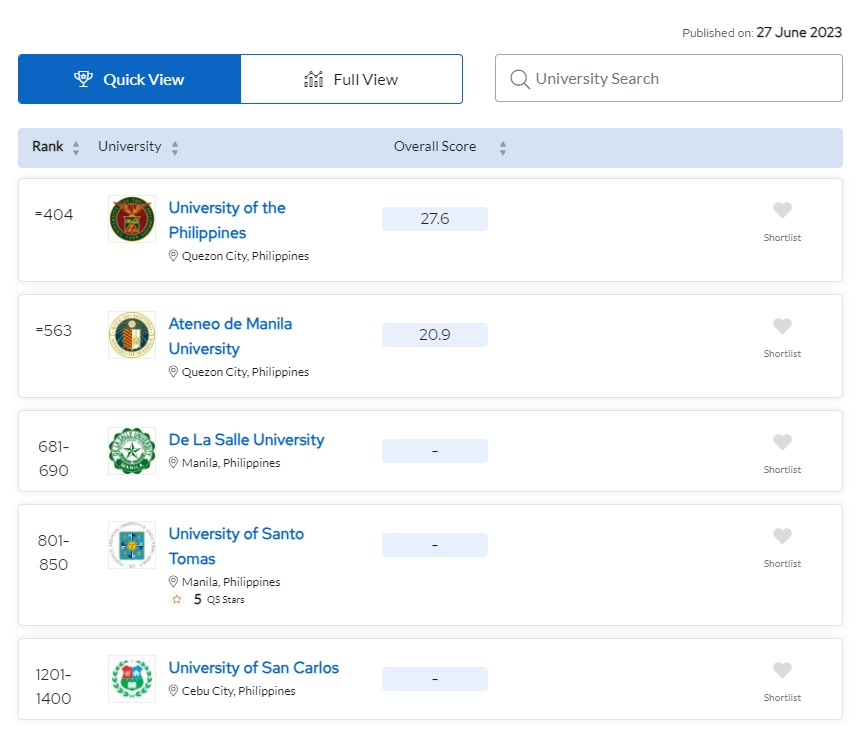Screenshot of QS World University Rankings featuring top universities in the Philippines. At rank 404, the University of the Philippines in Quezon City leads with an overall score of 27.6. Following at rank 563 is Ateneo de Manila University, also in Quezon City, with an overall score of 20.9. De La Salle University occupies the 681-690 range, based in Manila, though its score is unspecified. The University of Santo Tomas ranks between 801-850, located in Manila, with no overall score provided. Lastly, the University of San Carlos in Cebu City falls within the 1201-1400 range, lacking a specified score. Published on June 27, 2023, the ranking list includes features like quick view, full view, and a "University Search" bar. Each university entry is accompanied by a shortlist button, depicted by a heart icon.